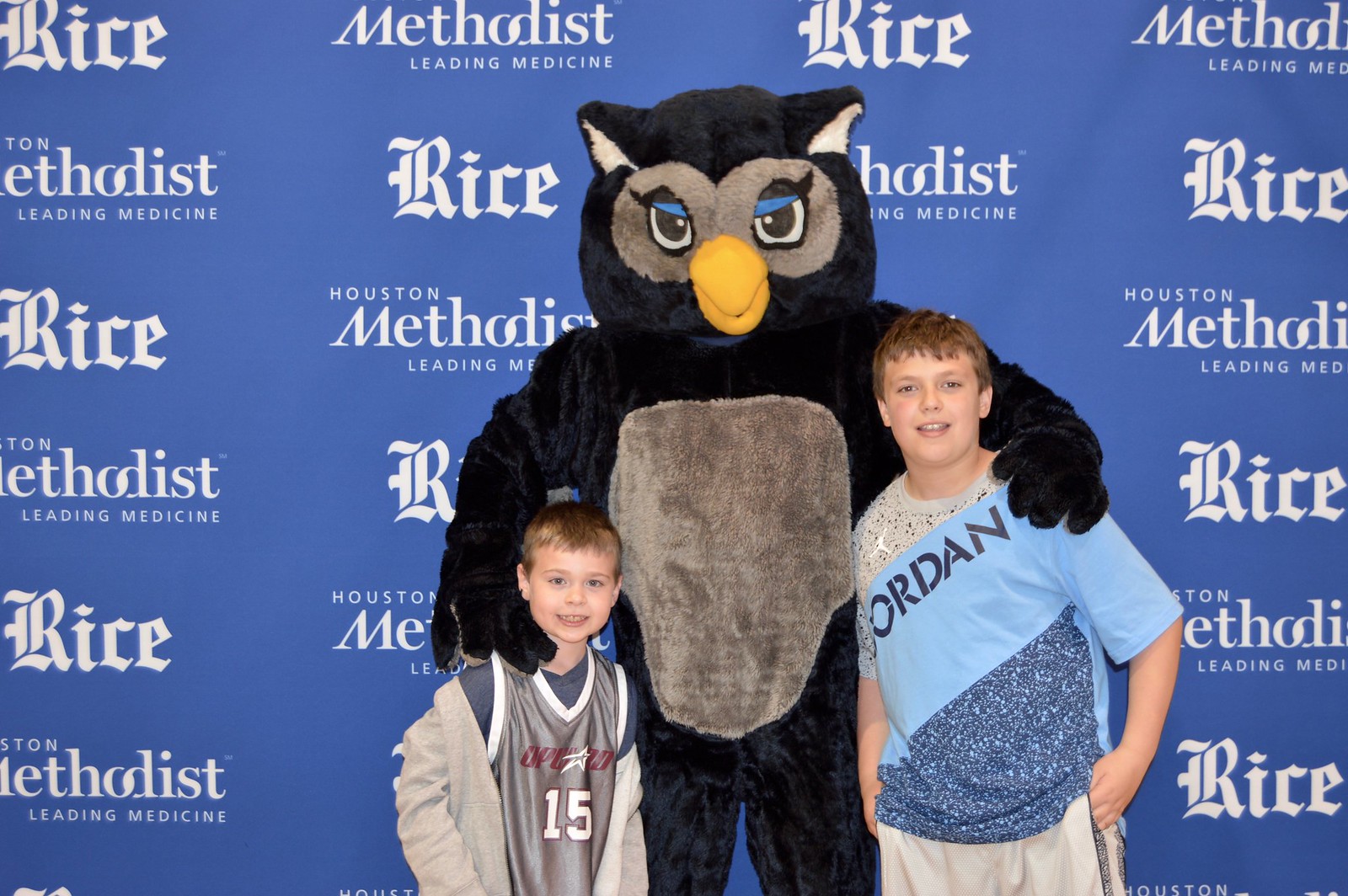In the image, a black and gray owl mascot stands between two white children, both with blonde hair, against a blue backdrop that features white text reading "RICE" in a Bavarian font and "Houston Methodist Leading Medicine." The child on the left, approximately six or seven years old, wears a basketball tank top with the number 15, over a darker blue-gray t-shirt and a gray sweatshirt jacket. The child on the right, around 10 to 12 years old, sports a blue t-shirt that says "Jordan" and gray pants. The younger boy beams with excitement while the older boy stands confidently, both reveling in the joyful moment with the captivating owl mascot.